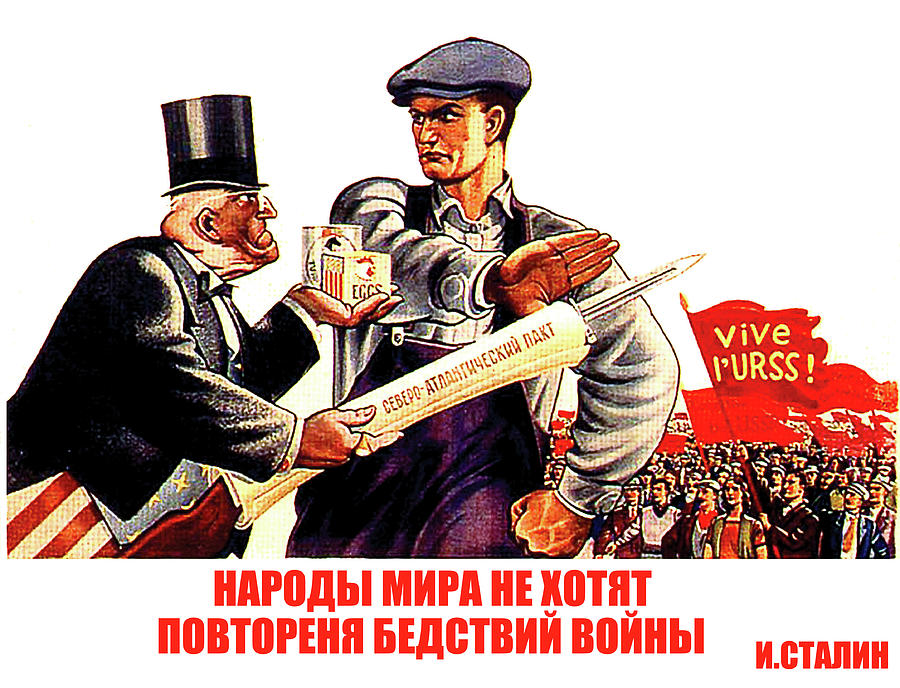This detailed and colorful political cartoon appears to be set during a protest in a foreign country, possibly Russia, given the elements and wording present. The scene is painted in a cartoonish style with vibrant hues and numerous characters. To the right bottom corner of the image, a crowd of people dressed in a variety of clothing, ranging from suits and ties to aprons, stands holding red flags inscribed with slogans like "VIVA IURSS." These flags underscore the collective protest theme. 

At the center-left of the illustration, an interaction between two main characters catches the eye. One man, resembling Uncle Sam with his quintessential red and white striped pants, a blue top hat, formal jacket, and glasses, is offering groceries, including a carton of eggs, to the other. This individual, depicted as a determined worker in a flat cap, suspenders over a white long-sleeve shirt, and overalls, is forcefully pushing away both the groceries and a weapon—a sword—Uncle Sam also holds. The worker's clenched fist and outstretched hand suggest a firm refusal.

Amidst this exchange, the background reveals a dense crowd of protesters, their red flags and unified stance highlighting a sense of solidarity and resistance. The bold red letters and the name prominently displayed beneath the two central figures add weight to the political message of the cartoon, echoing a common opposition to external influence and an unwavering stand for their cause.